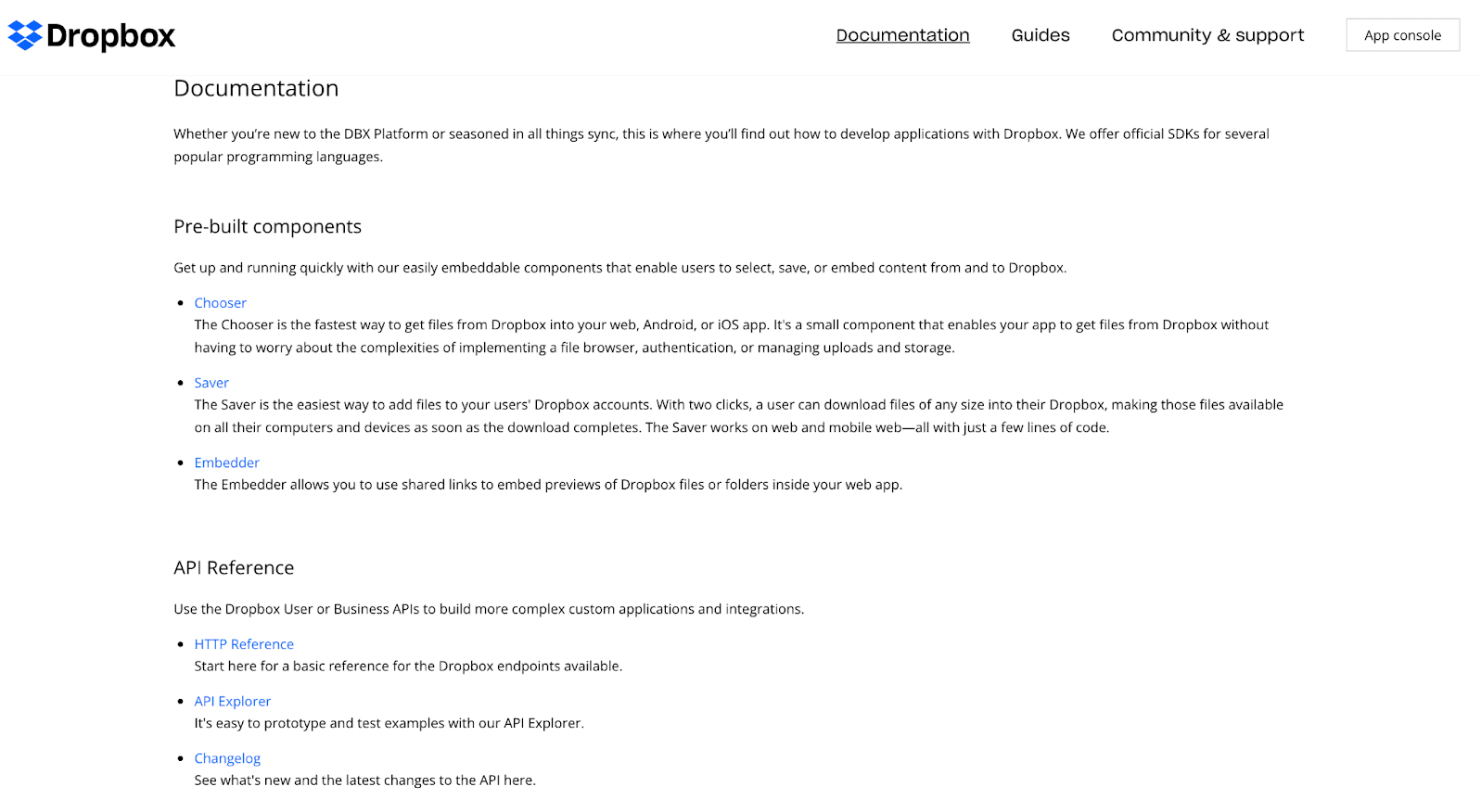This image is a screenshot featuring a white background and various elements organized in a structured layout. In the upper left-hand corner, there is a logo, followed by the bolded text "Dropbox" in black. Just right of the center, there is a navigation menu including options such as "Documentation" (underlined), "Guides," "Community," and "Support."

Below this navigation bar, aligned to the position where the word "Dropbox" ends, the title "Documentation" is displayed prominently in larger black letters. Beneath this title, there are two lines of smaller black text providing additional information.

Following approximately three lines of blank space, the heading "Pre-built Components" appears in black, succeeded by a descriptive sentence in black text. Underneath, there are three bullet points, each starting with a word in blue, accompanied by a line or two of explanatory text in black.

Further down, after more white space, the heading "API Reference" is displayed in black on the left side. Below this, there is a line of black text, and then another set of three bullet points. Each bullet point starts with a term in blue, such as "HTTP Reference," followed by a line of black text. This pattern continues for a couple more bullet points, each specified with different terms.